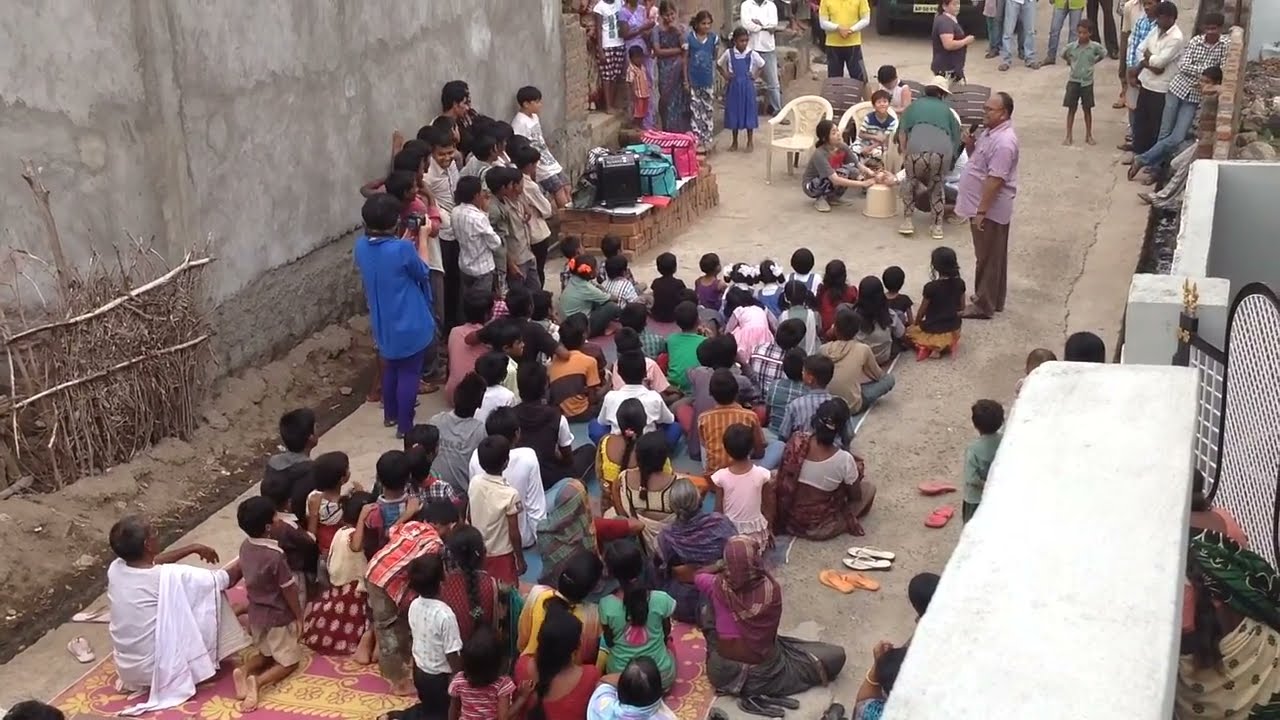The overhead image captures a bustling outdoor scene, possibly in a village setting, where a diverse crowd gathers on a paved but dusty road between two areas of buildings. The event appears to be a street play, with an announcer holding a microphone and giving instructions. Many people, dressed in vibrant colors including beautiful purple, pink, and blue dresses, are sitting on a rug placed on the ground, their sandals—orange, white, and pink—neatly set aside. The audience is varied, with men, women, and children ranging from the elderly to the young. Some spectators are seated in white chairs, while others stand on all sides, including against a cement wall to the left. Notably, some girls in blue dresses and a person in a yellow and white shirt are visible. In the background, clusters of people observe the scene, including someone squatting near a pottery area, appearing to craft pottery. The overall atmosphere suggests a lively community event.